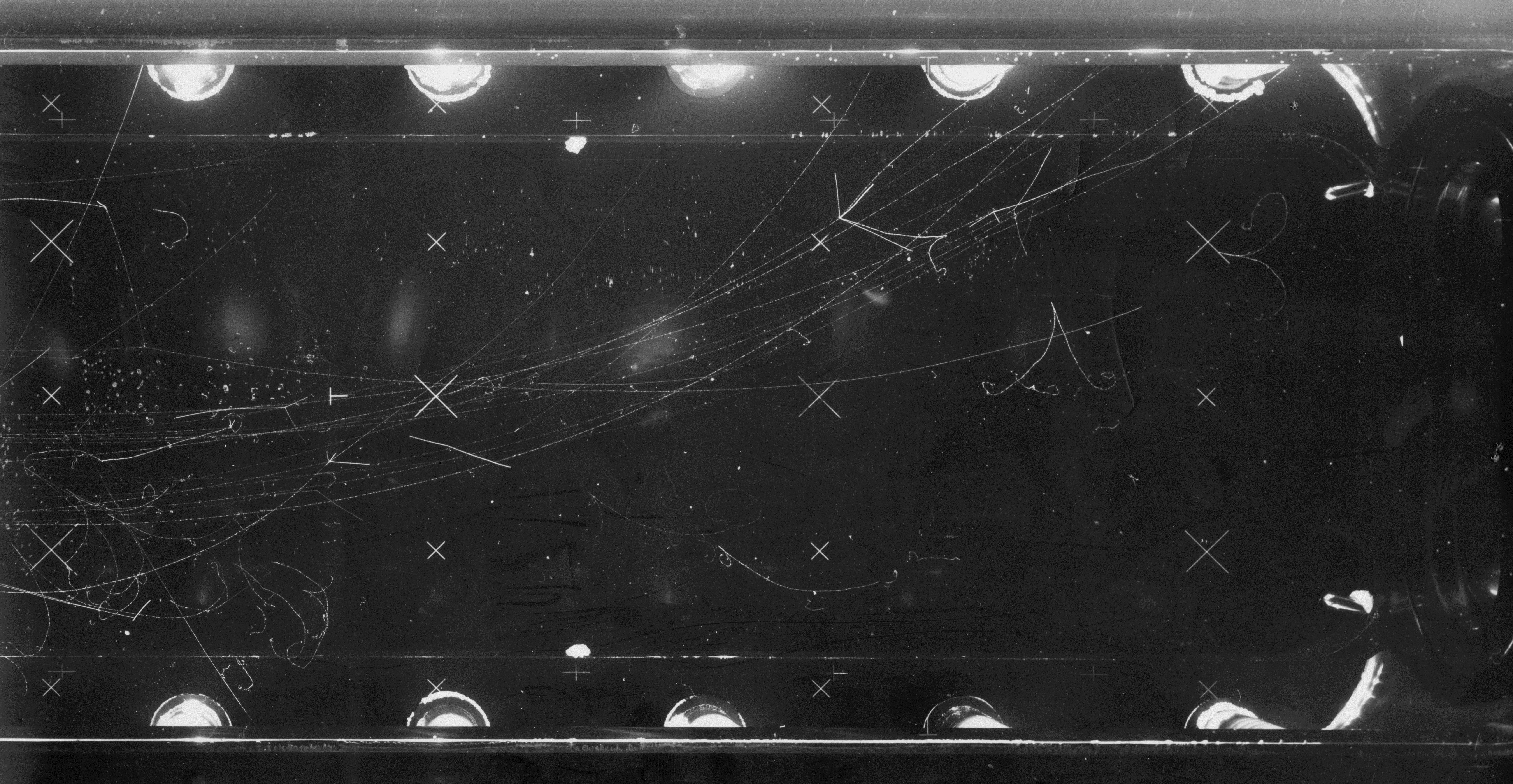Against a black background, the image is difficult to discern at first glance but reveals intriguing details upon closer inspection. The centerpiece appears to be a rectangular mirror framed by five light bulbs along both the top and bottom edges, resembling a dressing room vanity setup. However, the glass surface is heavily marred with numerous scratch-like marks, forming X's and curved lines that suggest broken glass. Some of these lines adopt a triangular pattern. Additionally, the image seems to contain some sort of reflective surface, capturing shadows of other lights, and there is a mysterious black oval to the side of the mirror. Overall, the image evokes an enigmatic, almost vintage quality with its grainy texture, and hints at a narrative of either plotting trajectories or simply the decay of a once-whole object now fragmented and obscure.